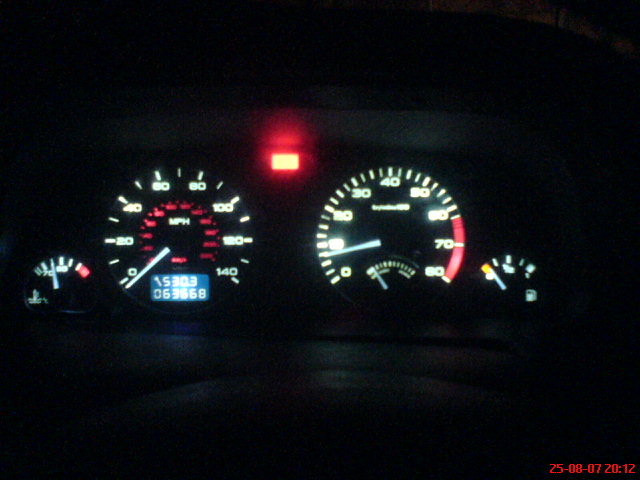A nighttime photograph taken from inside a car, captured with a camera as indicated by the red digital timestamp at the bottom right corner reading "25-08-07 20:12". The image focuses on the car's dashboard, showcasing various indicators. The fuel gauge is prominently featured, with the needle resting on 'E,' the empty mark, which is illuminated by a red warning light. The odometer displays a mileage of 63,668, indicating the car's usage. The temperature gauge is balanced in the middle, suggesting the engine temperature is optimal. The speedometer shows a slight movement, suggesting a speed between 8-9 miles per hour, though the image is slightly blurred, possibly due to motion or the camera flash reflecting off the dashboard.